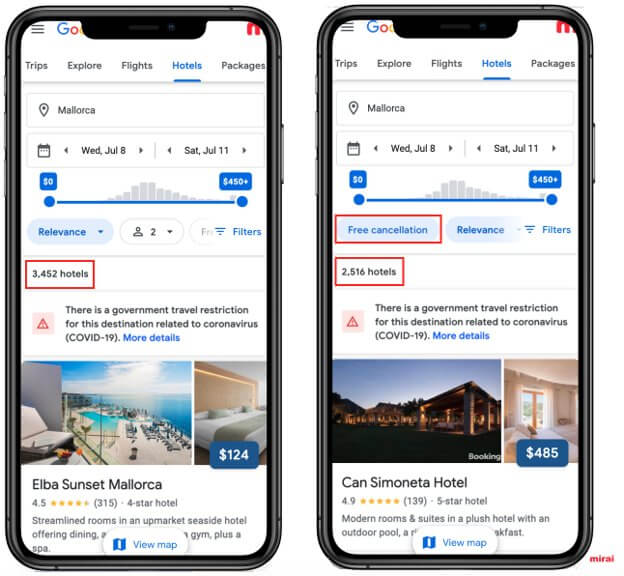The image captures two side-by-side mobile screens displaying Google search results for hotel bookings. Both screens prominently feature the Google logo truncated to "GO". At the top of each screen, a red home icon is visible on the right side, and three horizontal bars, indicating a menu, are on the left. The navigation bar above each screen displays options labeled: "Trips," "Explore," "Flights," "Hotels," and "Packages," with "Hotels" highlighted in blue and underlined, indicating the active selection.

Both screens show a search conducted for “Malacorsa” with dates specified from Wednesday, July 8th to Saturday, July 11th. Below the search bar, there is a price filter indicating a range from $0 to $4.50, visualized through gray bars that peak in the middle and taper at both ends.

Underneath, the left screen highlights "Rev Reveillance" with a note indicating free cancellation in a red box. It also states “3452 hotels” within another red box, while the right screen lists “2516 hotels” similarly outlined in red. 

A warning sign is present on both screens, warning about a government travel restriction for the searched destination due to coronavirus (COVID-19), with the note directing to "More details" in blue text.

The left screen displays a snapshot of the "Elba Sunset Mallorca" hotel priced at $124, whereas the right screen shows "Can Semineta Hotel" priced at $485. Additionally, the word "M-I-R-A-L" is seen outside the phone image on the right side.